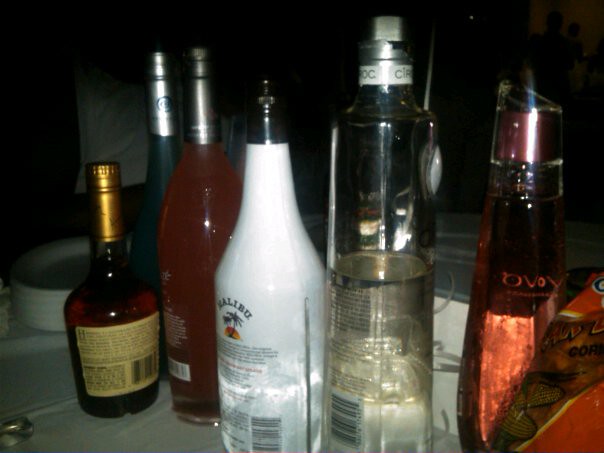This photograph captures a diverse liquor collection displayed on a white surface, likely a countertop. Centered in the image are six distinct bottles of alcohol. To the far left is a bottle of Hennessy, showcasing its characteristic golden-brown liquid and appearing unopened. Next to it is an opaque blue bottle, followed by a clear glass bottle containing a reddish-pink liquid. The fourth bottle is unmistakably a white Malibu bottle adorned with a palm tree graphic. Nearby, there's a clear bottle of Ciroc vodka, its contents half emptied. The lineup concludes with a clear bottle filled with a purple liquid. On the right edge of the photo, partly cut off, is a bag of orange-packaged chips. In the background, a stack of white Styrofoam plates and the suggestion of a faucet in the bottom left hint at a kitchen setting. The image is brightly lit in the center due to the camera's flash, leaving the edges darker and less detailed.